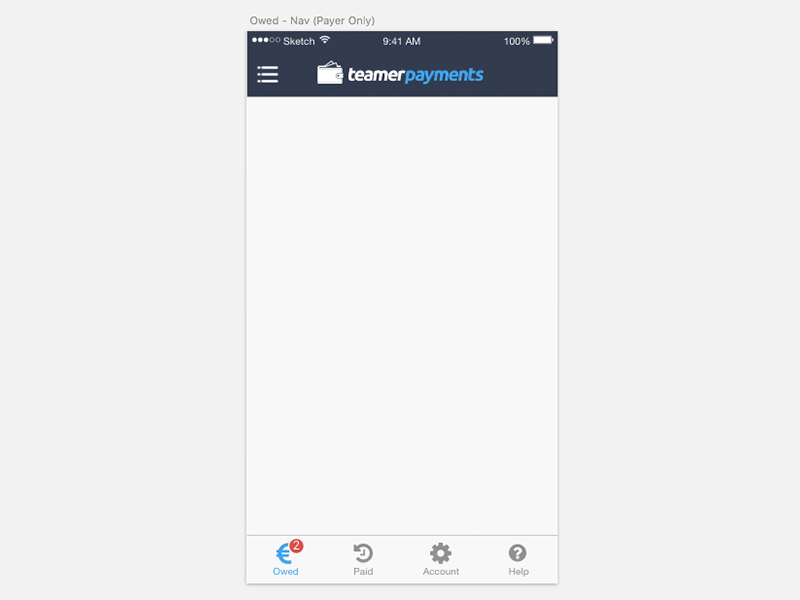The image depicts a screenshot set against a gray background. At the top of the screenshot, "Owed - NEF Payer Only" is prominently displayed. Below this, there is a navy blue rectangular section featuring a progress indicator with three out of five dots filled in. The status bar indicates the time is 9:41 AM, with a full signal and a 100% battery level.

In the middle section, three horizontal lines with small dots at their ends, resembling a menu icon, are present. Beside this icon, there is a file folder with documents protruding from it. The words "Teamer Payments" are written, with "Teamer" displayed in white and "Payments" in a lighter blue, all set against the navy blue background.

At the bottom of the screenshot, the interface contains several buttons. The "Owed" section is marked by a red circle with the number 2 inside it. Additional buttons labeled "Paid," "Account," and "Help" are also visible.

The image captures a detailed and organized interface design for a payment or financial application.